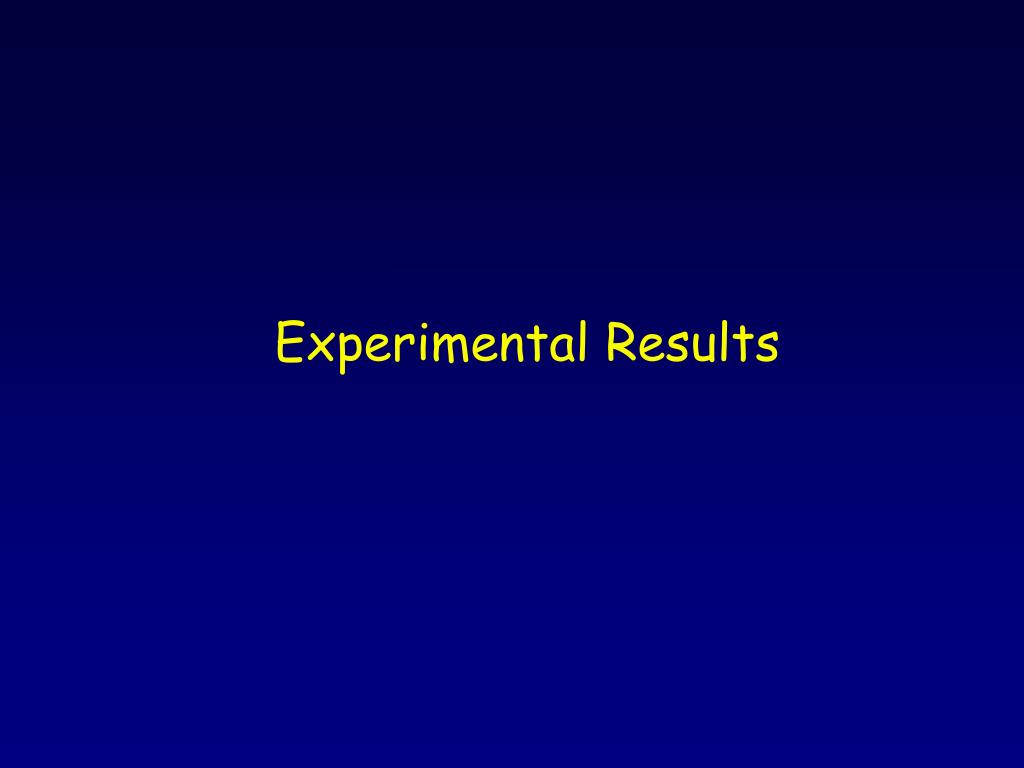The image appears to be a screenshot from a website or possibly a PowerPoint slide, featuring a visual labeled "Experimental Results." The background transitions in shades of blue, starting from a dark navy at the top, lightening to royal blue in the middle, and becoming the lightest blue at the bottom. The text "Experimental Results" is prominently displayed in bright yellow, with the letters "E" and "R" capitalized, while the rest are lowercase. The text is centered horizontally but positioned slightly above the midway point vertically. The font is sans serif and relatively small compared to the overall space. The visual does not include any additional graphics or elements.